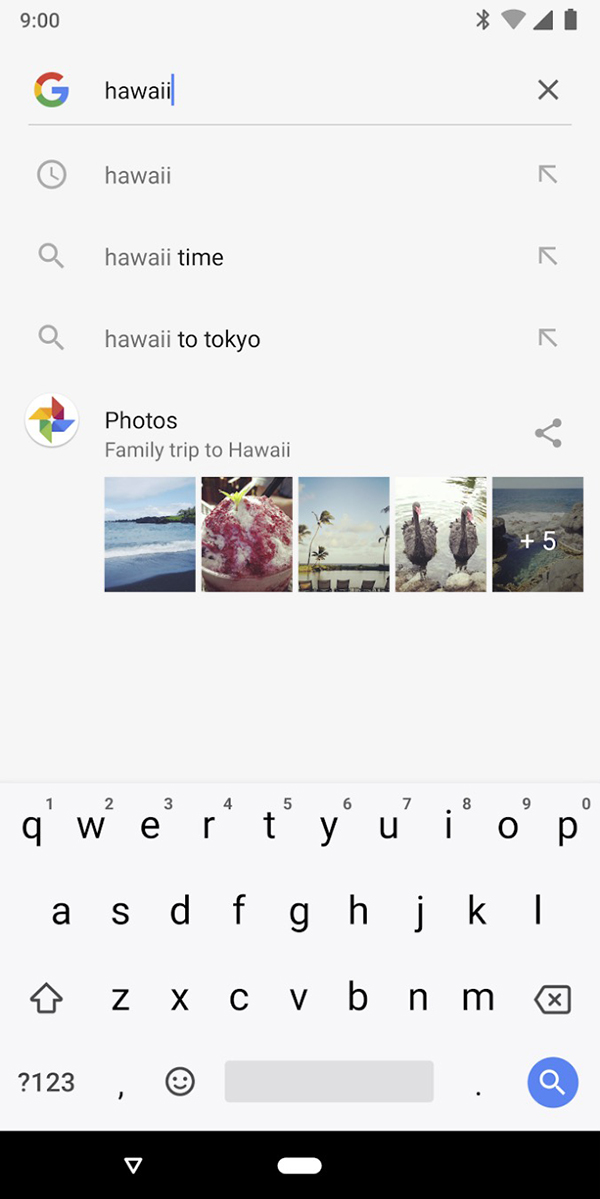The image features a user interface with a gray background. In the upper section, a clock symbol appears to the left of the word "Hawaii" which is followed by "9:00". This text is bold and is accompanied by "Hawaii" two more times below. A magnifying glass icon is situated to the left of each "Hawaii" text. Below, an arrow pointing diagonally up to the left accompanies each text.

Next, the interface shows a section labeled "Family Trip to Hawaii" with five photos displayed. The fifth photo is slightly grayed out with a "+5" in white indicating additional images.

Further down, there is a keypad layout featuring letters, an arrow, a house icon tipped to the left with an accent, a question mark, numbers (1, 2, 3), a comma, a smiley face, a space bar, a period, and a blue circle with a magnifying glass emblem. At the bottom of the screen is a black horizontal rectangle.

Overall, the image depicts detailed interface elements related to time zones, a family photo gallery, and a comprehensive on-screen keyboard.